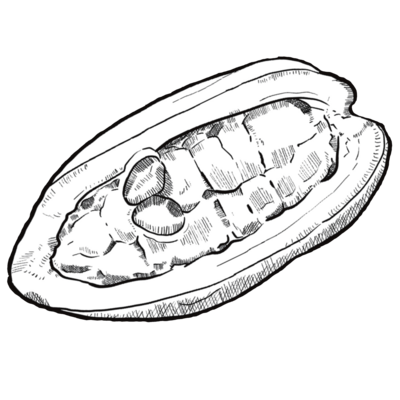This detailed black-and-white sketch depicts an elongated oval object, possibly a cross-section of a nut or kernel. The item is angled from the bottom left to the top right, with a dark, textured exterior and a lighter, segmented interior. The interior features two prominent rows of seeds or kernels, some round and others rectangular, shaded in gray. These seeds are reminiscent of corn kernels or teeth, adding to the ambiguity of the image. Two highlighted seeds stand out among the rest. The sketch combines elements of both natural and anatomical forms, evoking images of a grimacing mouth or a detailed botanical illustration. The background is stark white, offering no additional context or sense of scale, making the object appear isolated and somewhat abstract.